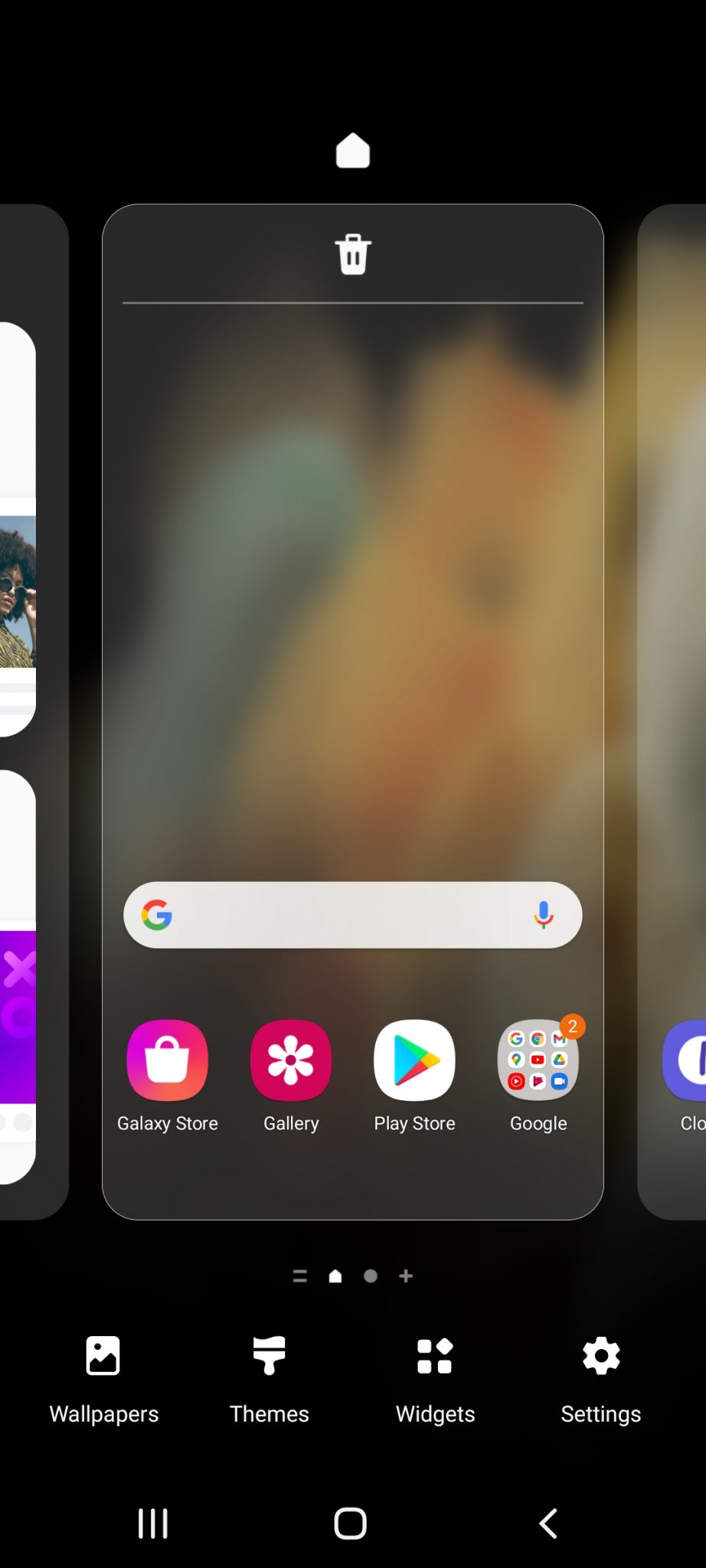The image features a screenshot capturing the screen of a mobile device set against a black background. At the center of the image is the outlined silhouette of the mobile device. The device's screen displays a slightly blurred wallpaper resembling flames in shades of blue, orange, and brown. Prominently positioned at the upper middle section of the screen is a large white delete icon.

Beneath the delete icon is a white Google search bar extending across the top portion of the screen, accompanied by a microphone icon on its right end. Below the search bar, four application icons are neatly aligned:

1. **Galaxy Store**: Represented by a white shopping basket icon set against a pink circular background.
2. **Gallery**: Illustrated with a six-petaled white flower on a round red background.
3. **Play Store**: Signified by a blue triangular play button on a white circular background.
4. **Google**: Indicated by the recognizable multicolored 'G' logo.

Each icon has its respective label written in white text directly below it.